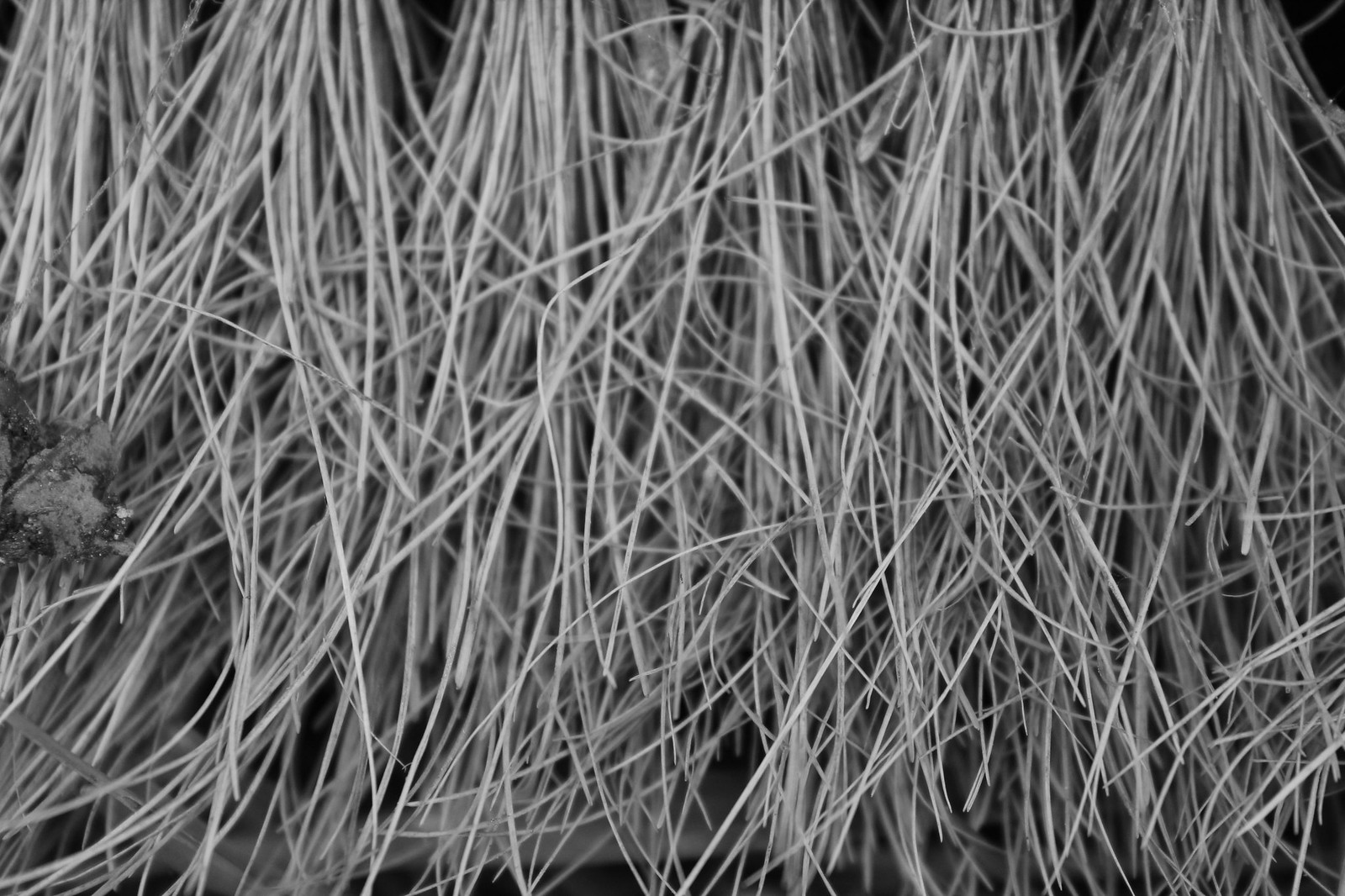The image showcases a detailed, black-and-white close-up of six bunches of hay or straw, arranged horizontally across the top. These bushels, starting narrowly from the top, fan out towards the bottom of the picture, creating an intricate web of tangled strands. The hay appears frayed and disheveled, some stray pieces jutting out at various angles. The entire scene is monochromatic, emphasizing the light gray hues of the fibrous material against the stark black background. Despite being tightly packed, the strands overlap and intertwine chaotically, filling the frame completely and adding texture to the composition. A small, indistinct area on the left adds a slightly different texture, perhaps indicating a denser clump or a different material, contributing to the overall complexity of the image.